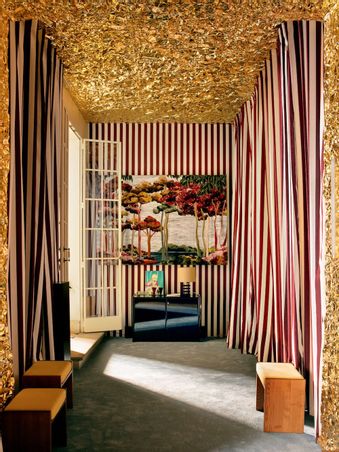The image depicts a long rectangular room or hallway with a luxurious and unusual design. The ceiling and walls are adorned with a shiny, speckled gold texture, adding a touch of opulence to the space. Along the length of the walls, there are vertically striped curtains in maroon, red, and white, creating a striking visual effect. Matching these curtains, the narrow back wall is also striped in a similar pattern.

At the center of this back wall, there is a large painting depicting yellow, green, and red trees. Below the painting sits a dark dresser, which is adorned with two lamps and a photo frame. To the left side of the room, there is an open French door with glass panes, allowing natural light to flood into the space.

The room is furnished with three small benches, colored in a brown and yellow scheme - two positioned along the left wall and one on the right. The floor of the room is gray, contrasting subtly with the rich colors above.